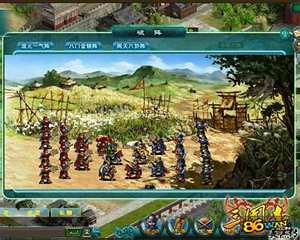The image displays a vibrant and detailed screenshot from a video game. In the foreground, numerous figures dressed in reddish and darker-colored clothes seem to be arranged in a formation, likely preparing for a battle. They stand on a patchwork of varying heights of green grass, with some small flowers scattered throughout. Wooden structures are noticeable, and the field transitions into rolling hills in the background. Above, a clear blue sky with fluffy white clouds sets a contrasting backdrop. 

The scene is further enriched with trees and a large building appearing in the secondary image beneath the primary one. Cartoon icons line the bottom of the screen, adding a playful element to the otherwise serious and strategic ambiance. The figures are positioned on a mix of brown dirt paths and grassy fields, reflecting an old-fashioned battle setting. The number 86 is prominently featured, though its significance is unclear. The image, which is relatively small in size (approximately 250 by 275 pixels), features a palette of blues, greens, and earthy browns with no discernible text in the immediate view.